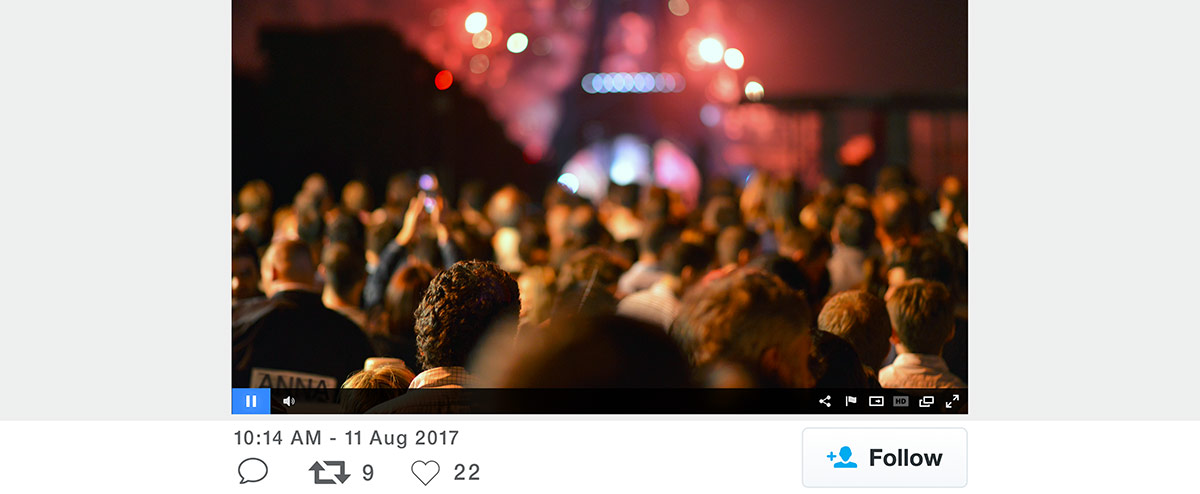Screenshot from an Unidentified Social Media Site: 

Central to the image is a vibrant photograph capturing a large crowd of people, all facing away from the camera, their attention riveted on the spectacle before them. The Eiffel Tower stands tall but blurry in the background, accentuated by numerous bright red fireworks that illuminate the scene. A considerable number of attendees are holding up their cell phones, evidently recording or taking photographs of the dazzling display. This image seems to serve as the thumbnail for a video.

At the bottom of the image, a black bar contains various interface icons indicating media controls: a pause icon on the left, a speaker/volume button adjacent to it, and on the far right, the share button, the flag button, and the full-screen option. Below this bar, the timestamp "10:14 AM, 11 August 2017" is displayed prominently.

Further down, the interaction buttons for the post appear: the reply button, the reblog/retweet button indicating 9 reblogs/retweets, and the heart button showing 22 likes. Adjacent to these buttons is a white rectangle with the word "Follow" in black letters, flanked by a blue icon of a person and a blue plus sign, inviting users to follow the content creator.

The entire image is bounded on either side by thick gray horizontal bars, framing the crowded scene and its digital interface neatly.